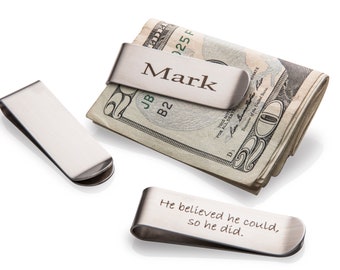The black-and-white photo showcases three distinctive silver money clips arranged on a pristine white background. The focal point is a money clip inscribed with the name "Mark" (M-A-R-K), securely holding a folded stack of $20 bills, with the denomination clearly visible at both the top and bottom edges of the folded bills. Positioned to the left, there is a plain silver money clip with no inscriptions. In the bottom right corner, another money clip is elegantly engraved in cursive with the inspirational quote, "He believed he could, so he did." Each money clip and the collection of bills cast a subtle shadow, emphasizing their presence against the stark background.